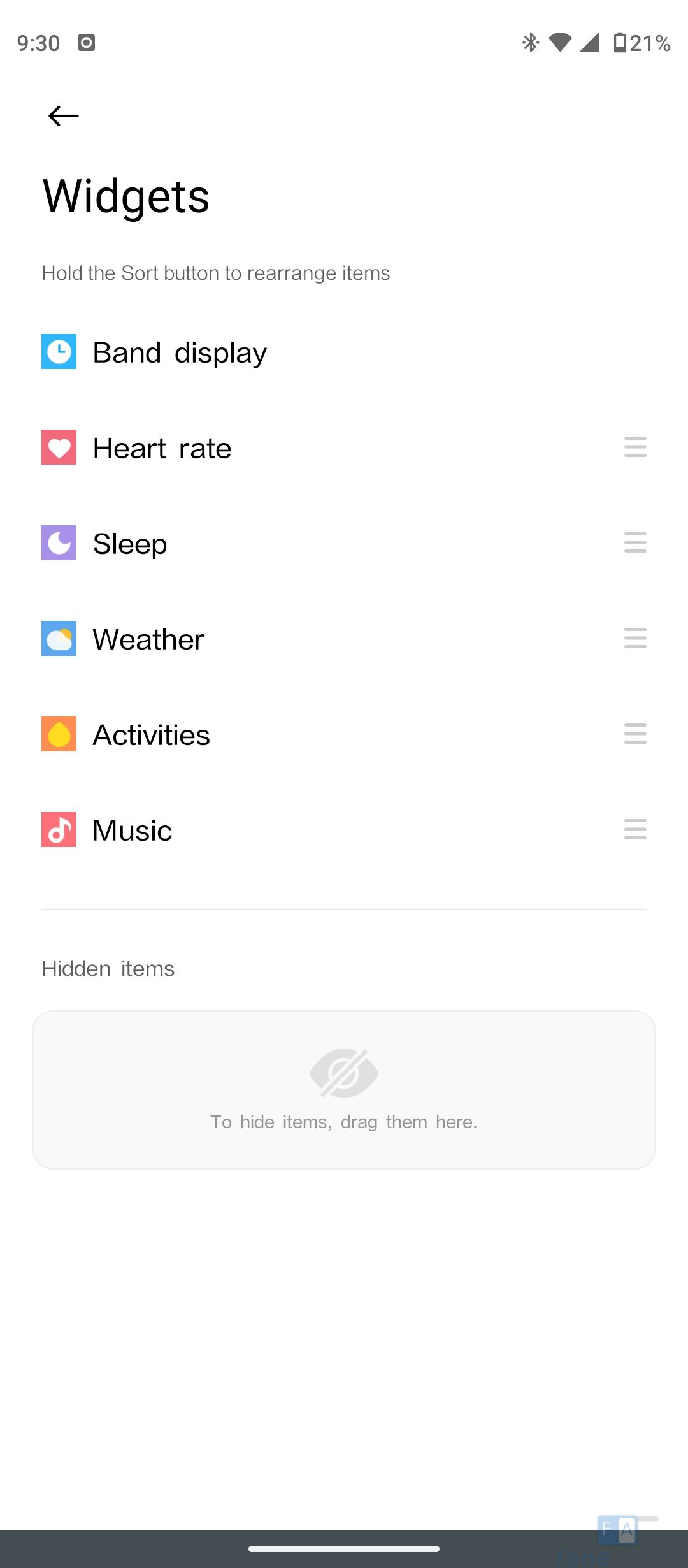In the upper left corner, the display shows the time as 9:30 in black text. To the right, there's the battery icon for the cell phone, positioned vertically with 21% remaining, indicated by the partially filled black section. Below this is a black left arrow.

Underneath the arrow, the word "Widgets" is displayed in capital letters, followed by the instruction "Hold the start button to rearrange items" in small gray text. 

The main section of the screen features several colored squares with white icons and text representing different widgets:

- A blue square with a white circle and the text "Band Display."
- A red square with a white heart icon and the text "Heart Rate."
- A purple square with a white moon icon and the text "Sleep."
- A blue square with a white cloud and yellow sun icon accompanied by the text "Weather."
- An orange square with the text "Activities."
- A red square featuring a white music note and the text "Music."

A couple of inches below this section, there's the text "Hidden Items" followed by a gray rectangle containing three lines. The instruction inside the rectangle reads, "To Redo Demo, Drag Them Here," repeated in gray text.